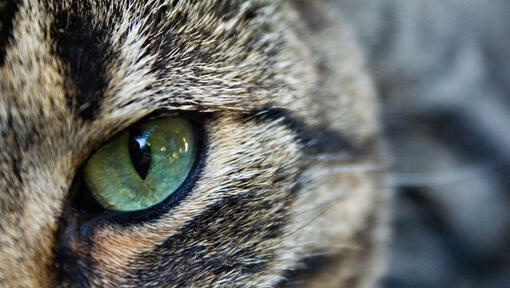The image is a striking close-up of a cat's eye, characterized by a mesmerizing green color with hints of yellow, brown, and hazel, and a distinct black, vertically-slit pupil. The photograph is horizontally oriented and predominantly captures the cat's facial features, with a sharp focus on the eye and the immediate surrounding fur. The fur exhibits a textured mix of colors, including dark brown, black, beige, and light tan, creating a marbling and striped effect that adds depth to the visual. The right side of the image is blurred, hinting at the cat's body or perhaps a gray striped design, with noticeable white whiskers extending from the eye area. This close-up composition emphasizes the captivating detail of the cat's eye, drawing immediate attention to its vibrant, almost jewel-like appearance.